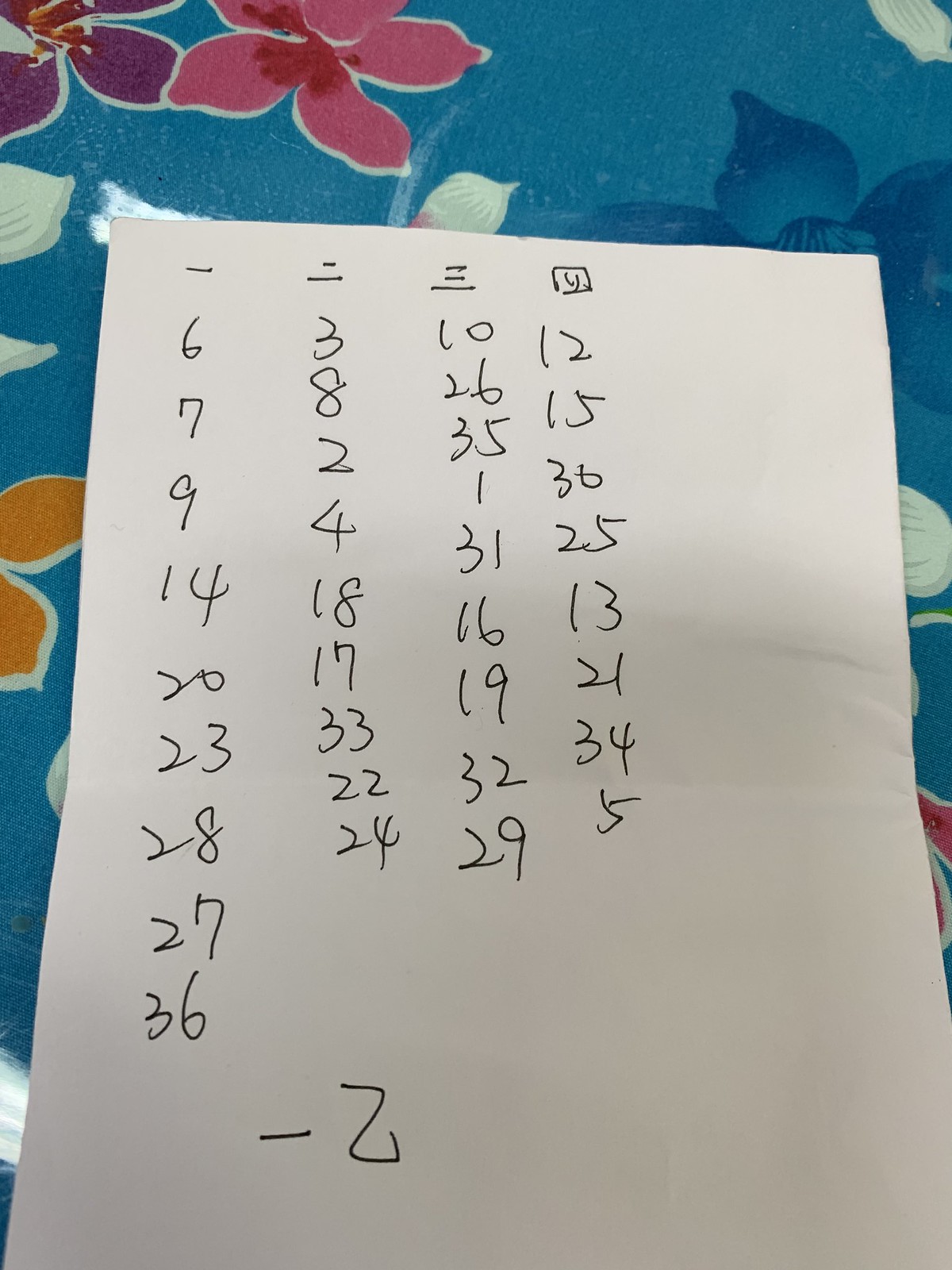A white sheet of paper is set against a vibrant, green fabric background adorned with various colorful floral patterns. On the paper, there are four columns filled with numbers written in no particular order. The first column displays the numbers 6, 7, 9, 14, 20, 23, 28, 27, and 36. The second column lists the numbers 3, 8, 2, 4, 18, 17, 33, 22, and 24. In the third column, numbers range from 10 to 29, and the fourth column features numbers ranging from 12 to 5, all in a random sequence.